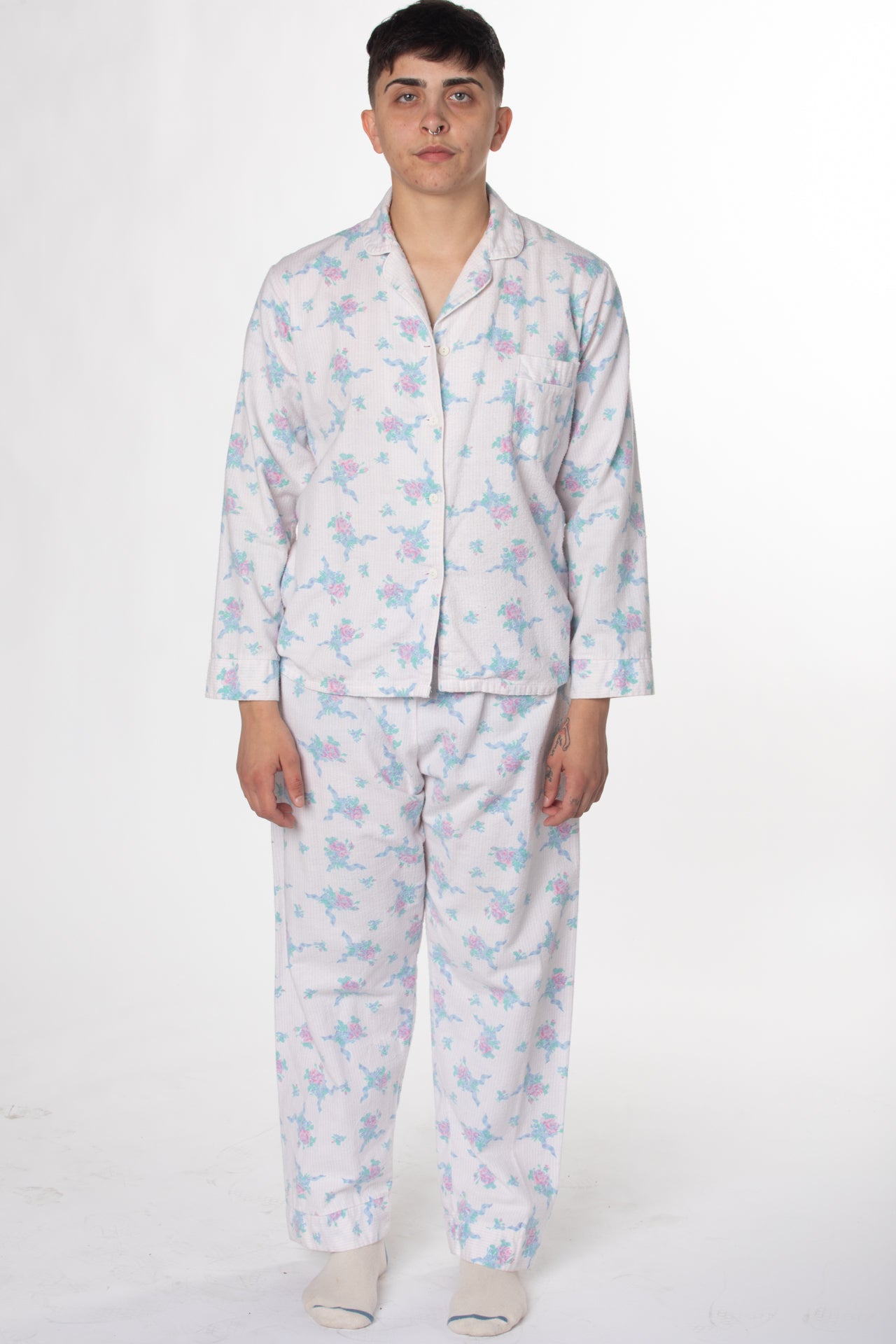In this image with a white to whitish-gray background, a young person stands centrally with their arms down at their sides. They have short black hair that's slightly longer on top but still above their eyebrows. Their facial expression is neutral. The individual wears matching white pajamas adorned with a pattern of purplish-pink flowers and green leaves, extending across both the long-sleeved top and the bottoms. These pajamas are buttoned down the front. On their feet, they wear white socks featuring a distinctive blue stripe, indicating where the toes should go. Additionally, the person has a nose ring and visible tattoos on their hand and fingers.